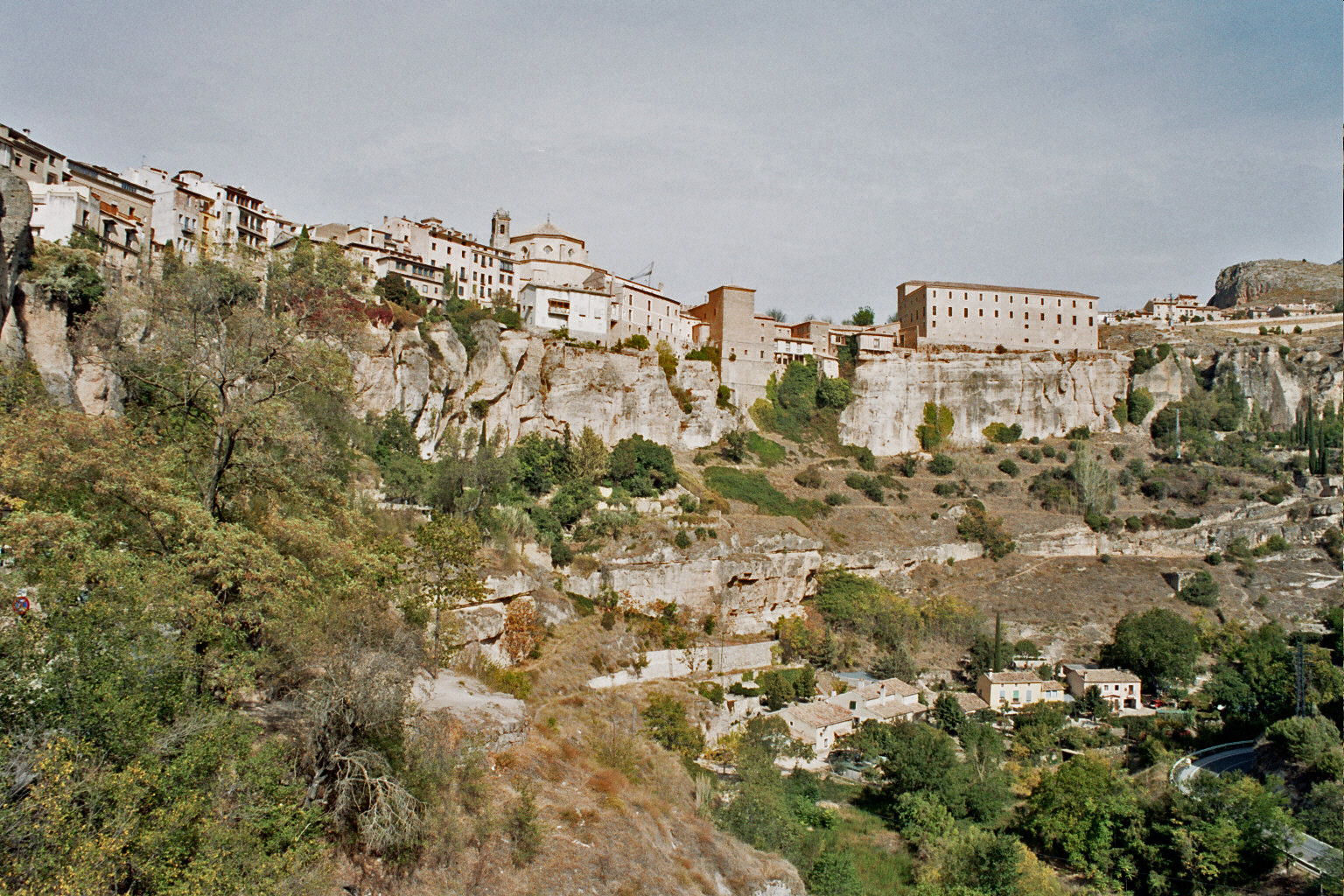This is a detailed photograph of a hill area taken from afar, which appears to depict an old city, potentially in Mexico, built on a ledge that descends into a slope. At the top of the hill, there are several large buildings and structures, while additional homes and man-made structures dot the slope as it cascades downward into the lower-right corner of the image. The hill is predominantly covered with lush green plants and trees, though some portions reveal brown patches of dried grass and plants, and parts of the rocky slope appear white. At the base of the hill, a canyon-like formation is visible, where the rocks have sheared off into the declivity. The sky above is a cloudy blue, adding to the atmosphere of the scene. This melding of natural beauty and aged architecture creates a picturesque landscape that is rich in historical ambiance.